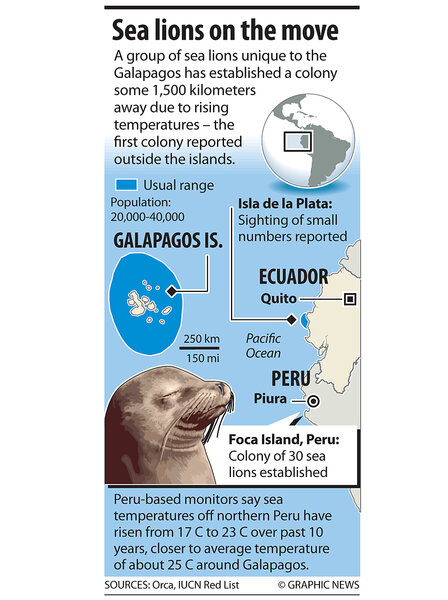The image is a vertical informational poster titled "SEA LIONS ON THE MOVE" in bold black capital letters. Beneath the title, it describes a group of sea lions unique to the Galapagos that have established a colony some 1,500 kilometers away due to rising temperatures. This is the first reported colony outside the Galapagos Islands. The poster includes a small depiction of a globe, highlighting the usual range of the sea lions, with a population estimated between 20,000 to 40,000. 

A blue box serves as a legend, indicating various data points, including a significant note on Isla de la Plata and sightings of small numbers pointing towards Ecuador and Quito. Another significant note marks a colony of 30 sea lions established on Foca Island, Peru. Detailed information at the bottom explains that Peru-based monitors have recorded sea temperatures in northern Peru rising from 17°C to 23°C over the past 10 years, nearing the average temperature of about 25°C around the Galapagos. 

The bottom of the poster credits sources such as ORCA, IUCN, Red List, and Graphic News. Finally, a small sea lion head with closed eyes is depicted in gray, enhancing the visual information provided.